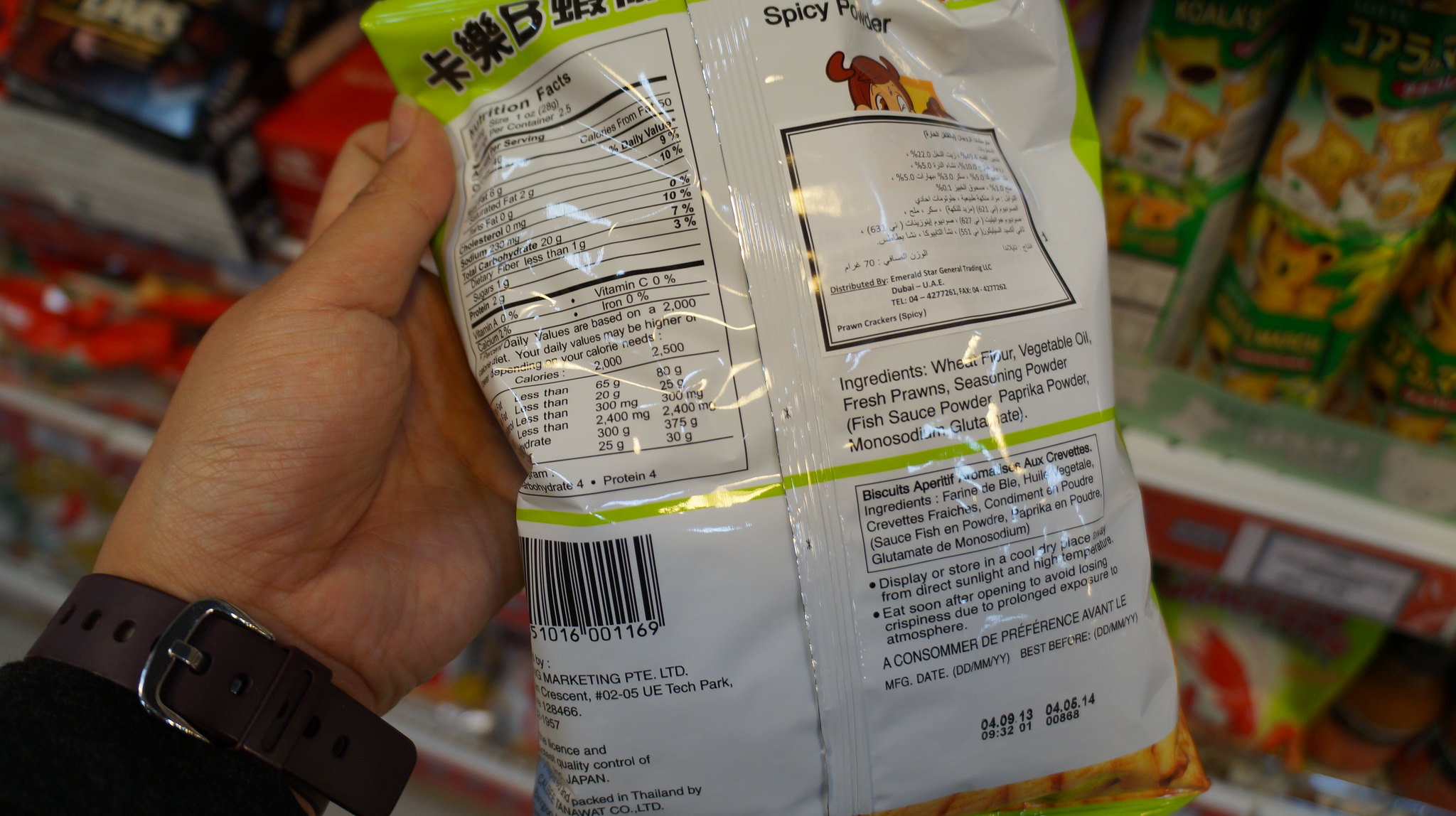In this detailed color photograph, likely taken with a GoPro or similar head-mounted camera, we see a snapshot inside a convenience store. The background is filled with blurred shelves stocked with various snacks and chips. Prominently featured in the foreground is a hand, specifically a left hand with a white but darker skin tone, appearing from the bottom left corner of the image. The person is wearing a brown leather watch with blue silver brackets and a black long-sleeved shirt. They are holding up a shiny foil bag of chips or snacks, displaying the back side of the packet to the camera.

The packet is notable for its reflective shine, which makes some details challenging to discern. However, we can see an imported Asian snack, likely from China or Japan, as indicated by square block letters on the packaging and a translated ingredient sticker. On the right side of the bag, the words "Spicy Powder" are visible, along with a list of ingredients including wheat flour, vegetable oil, fresh prawns, seasoning powder, fish sauce powder, paprika powder, and monosodium glutamate. Storage instructions and an urging to consume the contents quickly for optimal crispiness are also readable. The manufacturing date is marked as 4913, with a best before date of 4614. Additionally, the nutrition facts label on the left side is crumpled and mostly illegible.